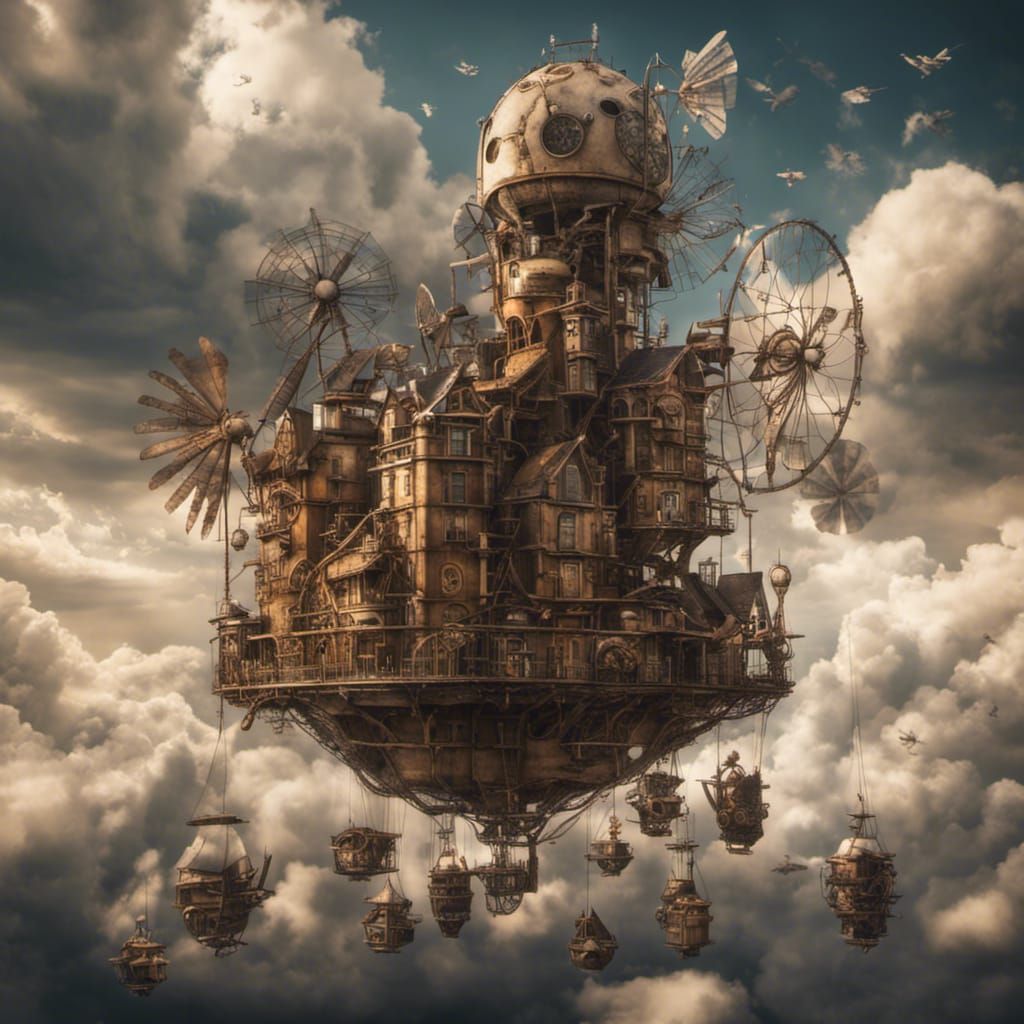This detailed rendering portrays a fantastical floating steampunk city predominantly colored in hues of brown, with minimal accents of white, tan, and cream. The city features numerous towering, multi-story Victorian-style townhouses, typically about four or five stories high. A large observatory dome stands atop, overlooking the intricate landscape. Scattered around the city are multiple windmills, some equipped with big fans and large gates or fences. The city lacks a visible propulsion system, but various parts of it hang down on ropes or wires, contributing to its eclectic and intricate design. Large birds glide through the sky in the upper right corner, where the thick, cloudy scenery clears up slightly, revealing a bit of blue. The overall composition includes small houses concentrated towards the lower center, enhancing the city's complex and layered appearance. In the backdrop, smaller steampunk-style aircraft can be seen navigating the fluffy clouds, adding depth to this imaginative aerial metropolis.